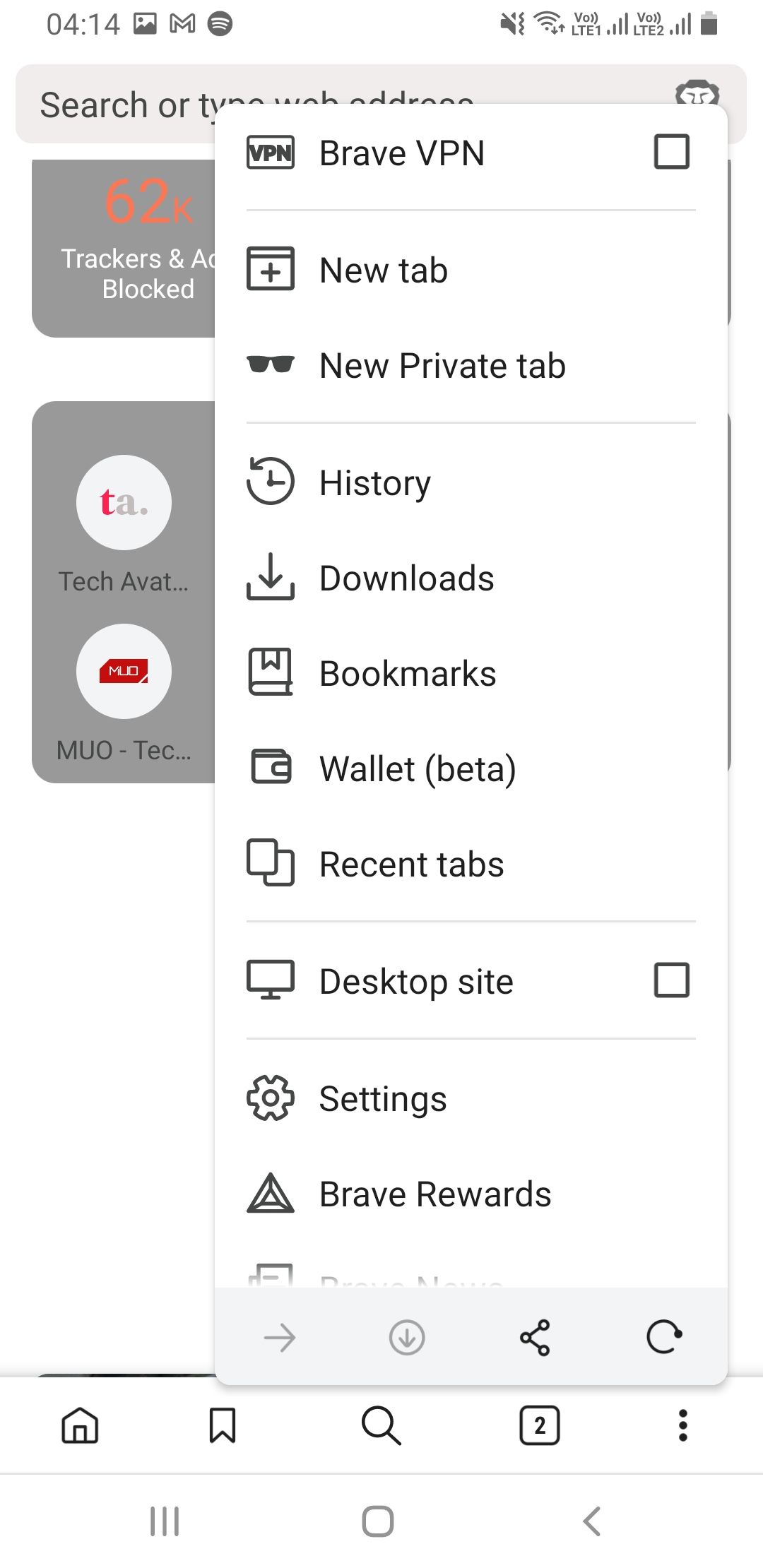Here is a cleaned-up and detailed description of the image:

---

This is a screenshot from a phone, showcasing a web browser interface. The right two-thirds of the screen is covered by a white pop-up tab. This pop-up extends from approximately half an inch from the top down to roughly one inch from the bottom of the screen. 

The upper part of the screen, behind the pop-up tab, features a gray search bar running across the width of the screen. In black text within the search bar, you can see part of the phrase "search or T," which is partially obscured by the pop-up. Above the search bar, there is a line of a white border containing a set of icons from left to right: 
- a clock showing the time 
- a picture icon 
- a mail icon 
- a circle representing the Wi-Fi icon 
- a battery icon 
- and a series of connectivity indicators showing full LTE signal on two connections, full Wi-Fi signal, and a muted sound icon.

Below the search bar, there's a dark gray rectangle displaying red text that reads "62 K." Beneath this, in white text, it says "trackers," then it continues under the visible area of the pop-up tab. There's a smaller white space present below this area, followed by another gray rectangle to the left containing a small gray circle with a red "T" inside it and a smaller gray dot nearby. Below this icon, there's black text that reads "tech at a V A T..." Additionally, there's a small white circle containing a red rectangle with "MUO" written inside it in white text. Below this in black text, it reads "MUO - TEC..."

The white pop-up tab itself has various elements: 
- At the top right corner, there's a white square with a black border.
- Below this, on the left side, there are icons matching with the following words to their right:
  - Brave VPN
  - New Tab
  - New Private Tab
  - History
  - Downloads
  - Bookmarks
  - Wallet (labeled as Beta)
  - Recent Tabs
  - Desktop Site (with another square icon on the right)
  - Settings
  - Brave Rewards

Underneath this list, there is a left-pointing arrow icon and a circular icon with a downward arrow. To the right of these, there are a share icon and a refresh button. Further down and to the left, there is a row of icons starting with a home icon, a bookmark icon, and a search icon. Additionally, there's a small white circle with a black border containing the number "2" in black text. On the far right side, there are three vertically aligned black dots, indicating additional options. 

Overall, this image captures a highly detailed view of the browser interface on a phone, highlighting various features and elements present on the screen.